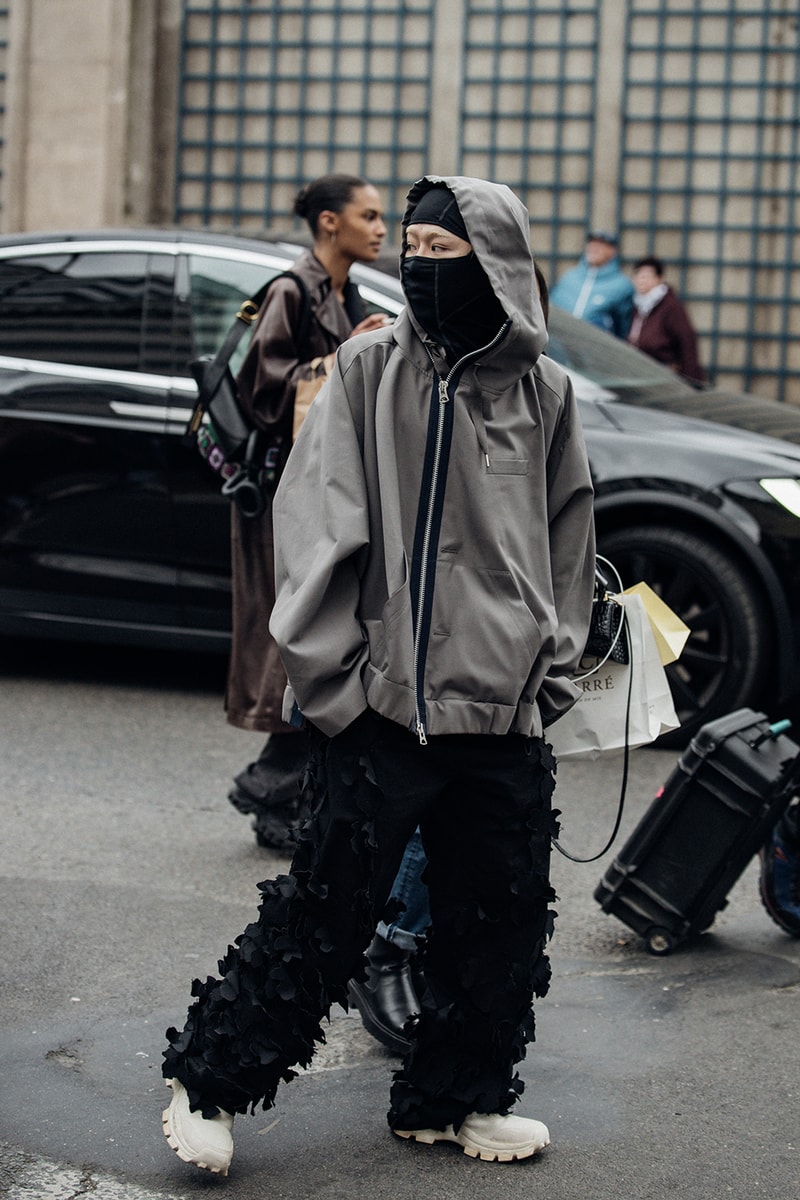In the middle of a street, a figure, possibly a girl or teenager, is captured walking in the front of the image. She is wearing an oversized gray zip-up jacket with a hood, reminiscent of a rain jacket, and an eye-cut black balaclava, giving her a ninja-like appearance. Her pants are striking, adorned from the ankles up with textured 3D flowers or ribbons, and she sports chunky-soled white tennis shoes. Behind her, there's a person partially visible in jeans and black boots, holding a bunch of bags and a purse. Surrounding them are several suitcases, and a black four-door sedan, possibly a Tesla, parked on the street. Further in the background, blurred, are two older individuals and a black car that could be indicative of a fashion shoot. Framing this outdoor scene is a solid tan building with a green trellis, adding to the urban backdrop.